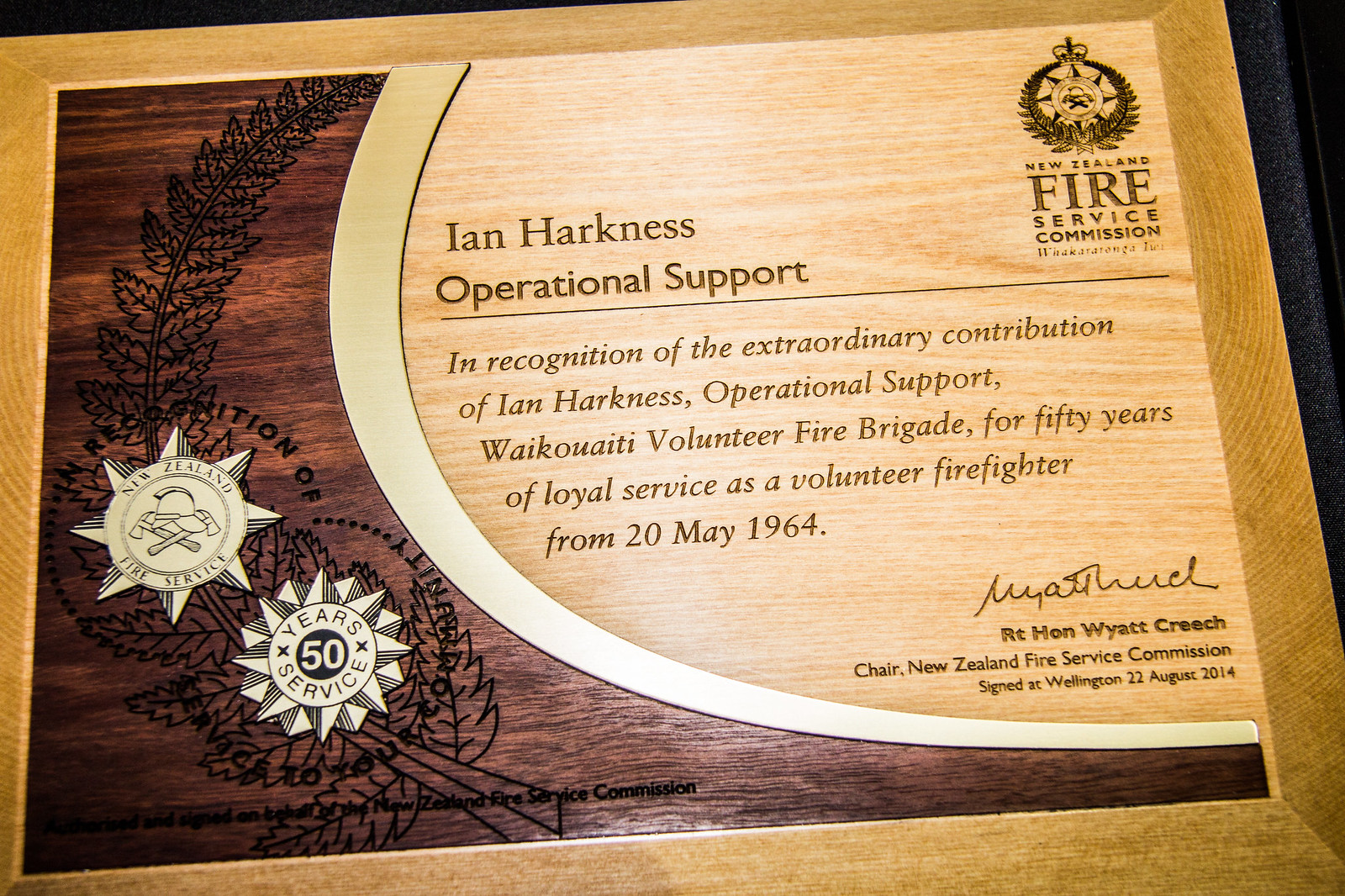The image is a photograph of a wooden plaque, beautifully crafted with a detailed wooden frame that has a light brown, almost beige, rectangular border. The interior of the plaque features varying shades of brown wood, showcasing intricate etching. On the left-hand side, there is a darker wood area with a black leaf background, against which two medallions are prominently displayed. The top medallion reads "New Zealand Fire Service," while the one below it commemorates "50 years of service." The primary body of the plaque highlights in yellowish-brown lettering: "Ian Harkness Operational Support." Below this, an inscription reads: "In recognition of the extraordinary contribution of Ian Harkness Operational Support, Wakawati Volunteer Fire Brigade for 50 years of loyal service as a volunteer firefighter from 20 May 1964." In the top right corner, there is another medallion with the text below it stating "New Zealand Fire Service Commission." At the bottom right of the plaque, there is a signature that reads "RT Honourable Wyatt Creech, Chair New Zealand Fire Service Commission, signed at Wellington, 22 August 2014."